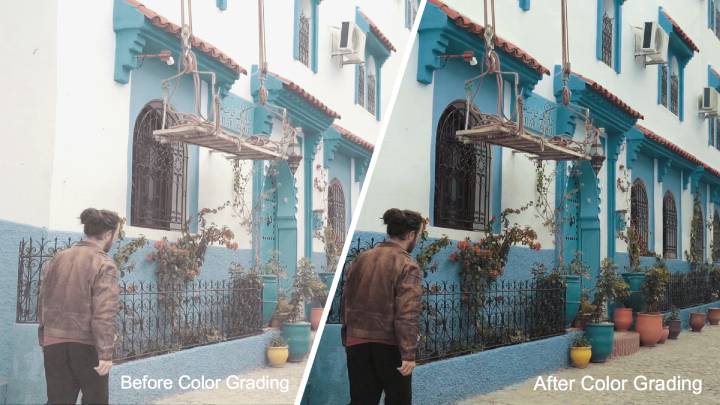This image showcases a side-by-side comparison of a photograph before and after color grading, divided by a diagonal line slanting towards the top right. On both sides, the picture features a house with white exterior walls accented by vintage architectural windows with blue borders and an air conditioning unit mounted on the facade. Below the windows, there are flower pots of diverse colors and a small garden area encircled by a railing. A man with black hair tied in a bun is depicted walking in front of the house, dressed in a brown jacket and black pants. The left side of the image is labeled "Before Color Grading" and appears less vibrant, with the white walls looking overexposed and the blue sections appearing muted. On the right side, labeled "After Color Grading," the same scene appears more vivid and detailed, with enhanced saturation and contrast making the colors of the house, the man's clothing, and the surrounding plants look richer and more distinct.